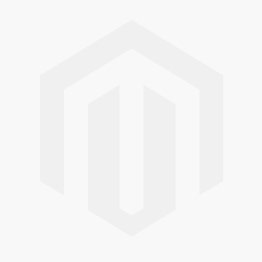The image is a square, full-color photograph with no border. It depicts a neon-like, minimalist representation of a car in glowing orange and dark orange lines, which gives the impression of a heated or fiery effect. The car, seen in its general shape with visible wheels, windows, and bumper, is set against a predominantly grayish background, which fades from whitish at the top to a more defined gray. At the bottom of the image is a distinctive white or gray vent with vertical slashes and a solid base. The car is centered and slightly diagonal, descending towards the right. There are no people, animals, or text in the photograph.